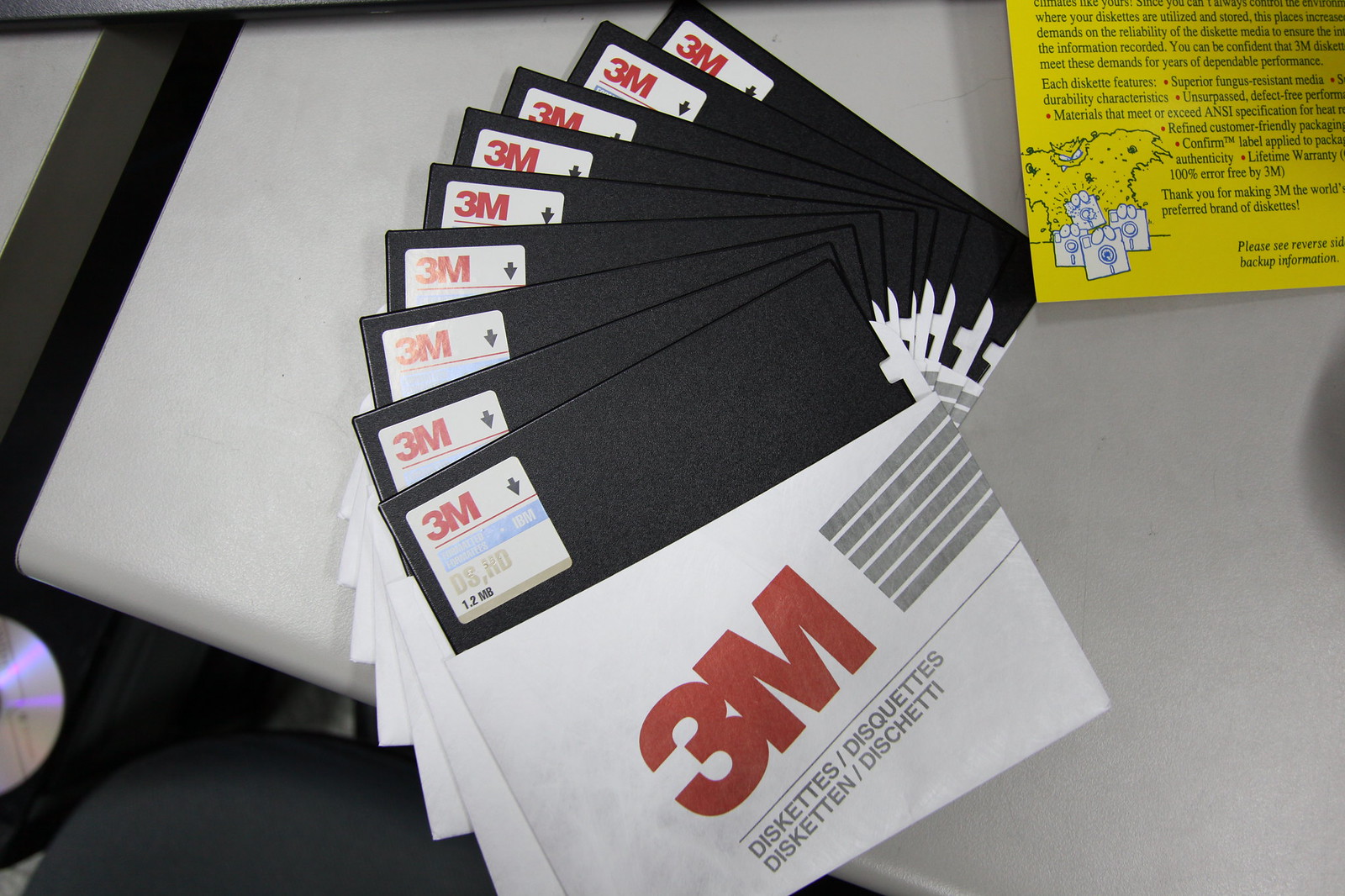The photograph features nine 5 1⁄4 inch floppy disks made by 3M, fanned out in a spiral on a plain white table. Each disk has a black top and a white bottom, with the 3M logo prominently displayed in red text on a sticker located on the top left corner of each disk. The disks are labeled "DS HD" indicating they are double-sided and high-density, likely with a storage capacity of 1.2 MB. The background includes the edge of a chair and possibly a part of a computer case with a silver CD on top, as well as a yellow piece of paper in the top right corner, featuring a lot of text and a cartoon drawing of a monster discussing the features of these floppy disks.